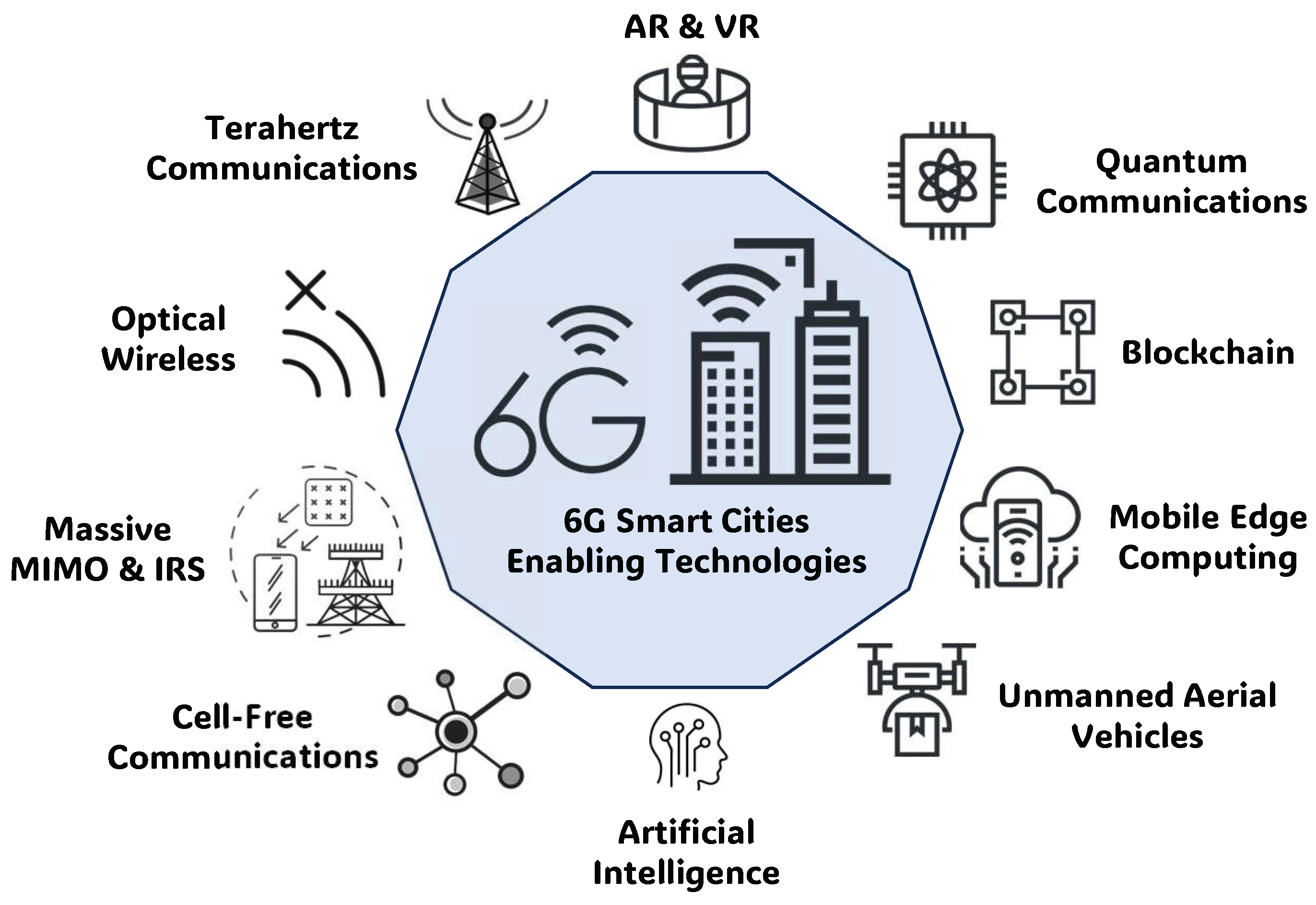The image is a detailed diagram on a white background outlining 6G Smart Cities Enabling Technology. At the center is a light blue octagonal shape labeled "6G Smart Cities Enabling Technology" in black lettering. On the left side of this shape, there's a "6G" sign accompanied by three inverted arcs resembling a computer signal icon. Flanking the central shape are two tall buildings displaying these signal arcs, symbolizing connectivity.

Surrounding the main octagon, the diagram contains various symbols and descriptions of the technologies enabled by 6G. At the top, it features "AR and VR" with a corresponding symbol. The technologies are listed clockwise and include: quantum communications, blockchain, mobile edge computing, unmanned aerial vehicles (UAVs), artificial intelligence (AI), cell-free communications, massive MIMO and IRS, optical wireless, and terahertz communications. Each of these technologies is annotated with unique symbols, making the diagram easy to follow and comprehensive in highlighting the components of 6G urban infrastructure.